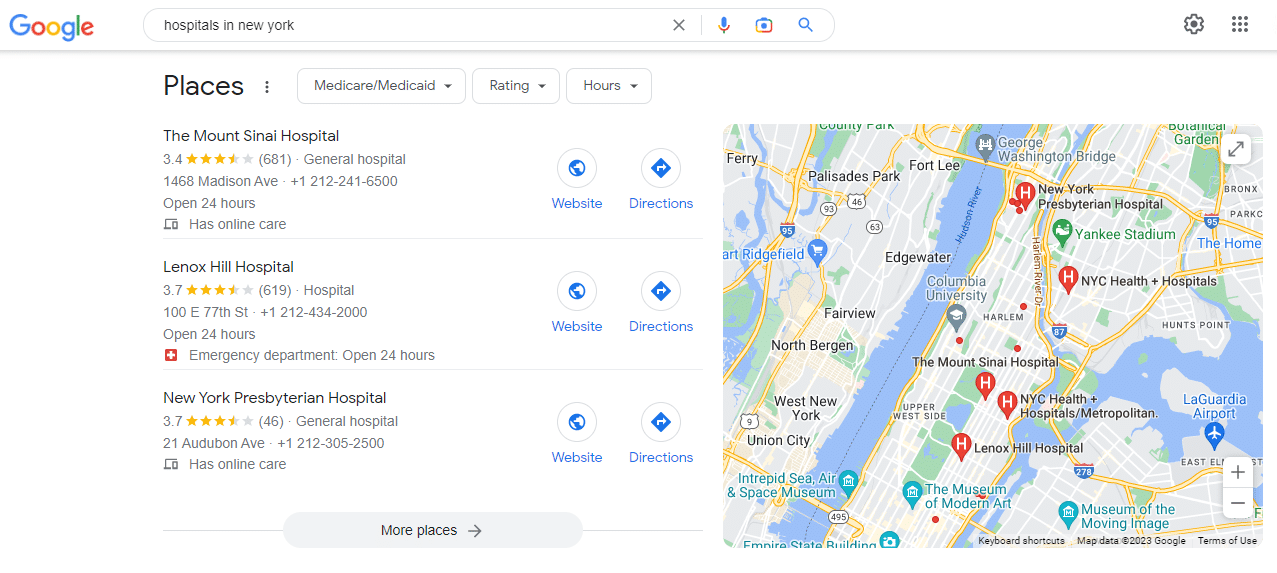This screenshot showcases a Google search results page for "hospitals in New York." The interface displays the typical Google search features, including, from left to right: an 'X' to clear the search, a microphone icon to enable voice search, a camera icon for image search, and a magnifying glass to initiate the search. To the far right, there is a cogwheel for settings and a grid of dots representing additional Google apps.

Below the search bar, there's a sorting section labeled "Places" with options to filter results by features like Medicare, Medicaid acceptance, ratings, and hours of operation through a menu of three dots.

The search results feature three hospitals:
1. **Mount Sinai Hospital:** This general hospital has a rating of 3.4 out of 5 stars.
2. **Lenox Hill Hospital:** This facility boasts a 3.7 out of 5 stars rating and offers a 24-hour emergency department.
3. **New York-Presbyterian Hospital:** Also rated 3.7 out of 5 stars, this hospital provides online care.

Each hospital listing includes buttons for accessing their websites and obtaining directions. Additionally, users have the option to view more places related to the search at the bottom of the listed hospitals.